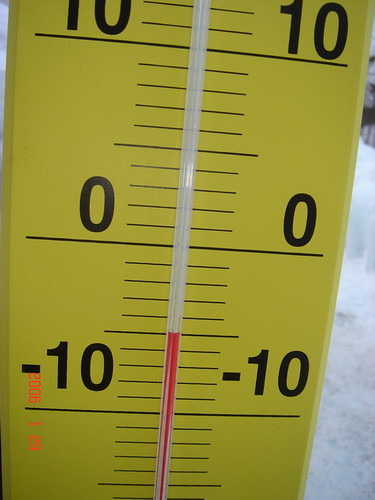The image is a close-up photograph of a thermometer taken with an old digital camera, evidenced by the vertical orange date stamp on the left side, which appears to partially read "2006." The thermometer itself is a traditional, vertically-oriented design with a yellow background, black lines, and numbers marked in increments. The red mercury line inside the thermometer indicates the temperature, which is currently between -8 and -7 degrees Fahrenheit.

On the right side of the image, there is a thin sliver of white, suggesting a large amount of snow, and at the top of this white area, something resembling railings is visible, adding context to the outdoor setting. The thermometer's close-up view prominently displays the range from -10 to 10 degrees Fahrenheit, with additional markings extending down to -20 degrees. The scene captures a frigid winter day, with snow accumulation high enough to obscure part of the background.